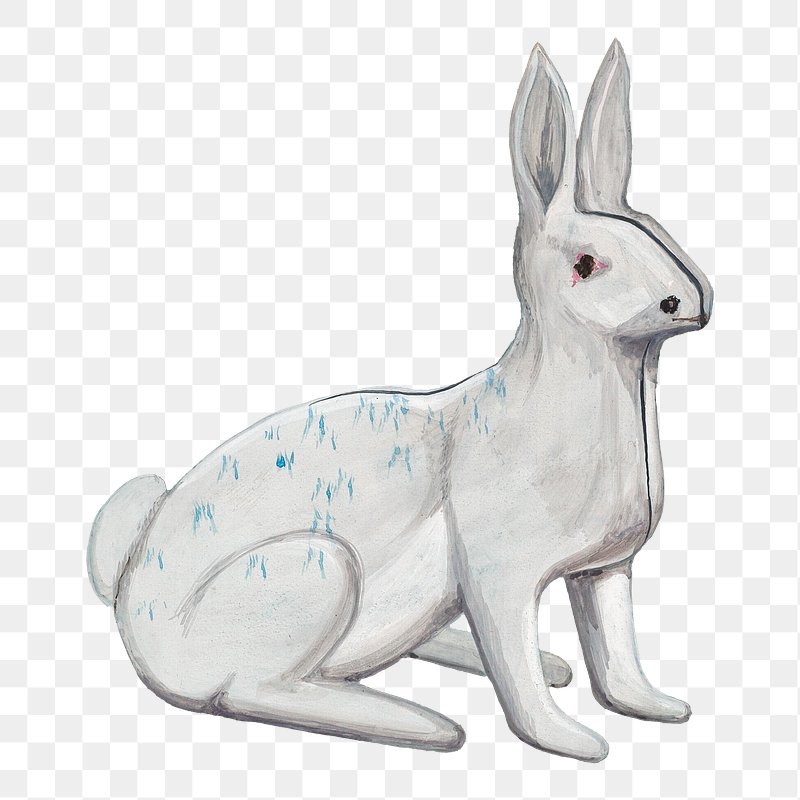The image is a stock illustration suitable for web pages, featuring a detailed, almost toy-like white bunny rabbit with a checkered background. The background consists of a gray and white checkered pattern that fades to a lighter shade towards the bottom. The bunny is depicted as a drawing or painting and is positioned in the foreground, occupying most of the 29 rows of the checkered backdrop. The bunny is in a seated position, facing to the right, with upright, attentive ears. It has observable seams down the middle of its face and front body, contributing to a toy-like appearance. Its eyes are black with rusty hues around them, and there is a little pink around its visible eye due to the profile view. The bunny’s nose is a prominent black dot, and its cottontail is distinctly visible. Additionally, the bunny features small blue markings on its back and one of its legs, further enhancing its detailed design. The overall expression of the bunny is neutral, not conveying any specific emotion.